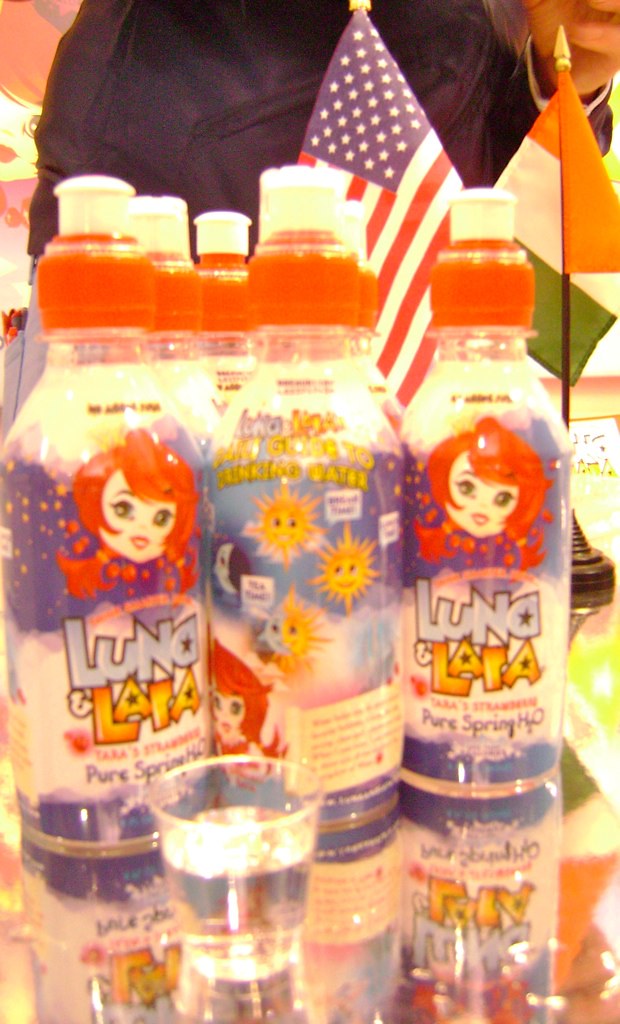In a brightly lit indoor setting, this vertically rectangular image depicts a shiny, mirror-like countertop reflecting several items. Central to the image are three bottles of Luna and Lara Pure Spring H2O, standing upright side-by-side. The bottles feature a colorful, cartoonish design of a smiling woman with red, wispy hair and red lipstick. Prominently displayed on the bottles are the brand names "Luna" in blue and "Lara" in reddish-orange, along with the text "Pure Spring H2O" in blue and yellow. Each bottle is topped with a white squirt cap and a red plastic cap below it. In front of the bottles, a clear plastic sampling cup filled with water sits on the counter. Flanking the setup, small American and Irish flags are mounted on thin black poles, adding a patriotic and international flair to the scene.